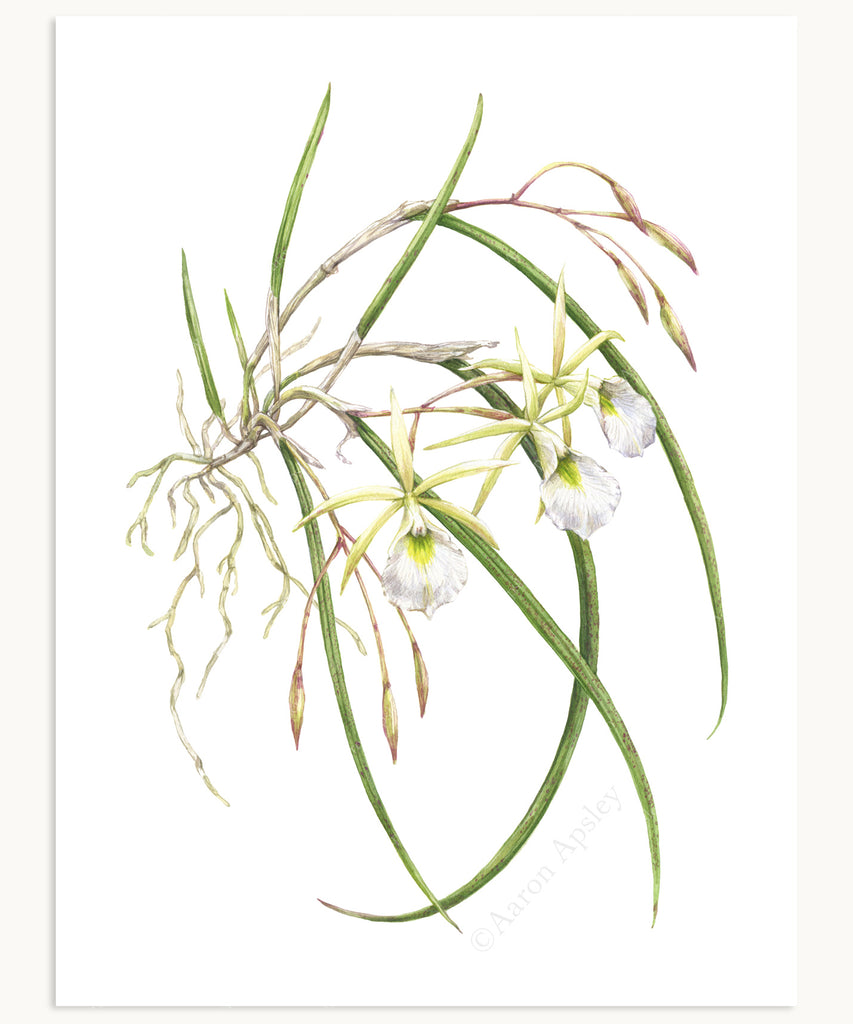The image depicts a detailed color drawing of a plant, set against an eggshell white background. The rectangular canvas, measuring approximately five to six inches high and four to five inches wide, showcases the plant's extensive root system prominently on the left-hand side. The roots are thin tendrils that appear to suspend the plant in the air. The plant itself features long, thin leaves that grow upward and around, starting from a white, papery base before extending into green foliage. Each leaf measures about an eighth of an inch wide and three to four inches in length. 

In the center, the plant boasts three distinctive flowers with large, tubular white petals. One side of each petal lowers, revealing a yellow and green interior base. Beneath each flower, five pointed leaves fan out in a starfish shape, exhibiting a light yellow-green hue. The shadow effects in light gray are visible along the left-hand side and bottom of the canvas, adding depth to the image. 

The overall visual presentation is vibrant, with a clear, bright setting and a palette that includes shades of green, light green, brown, and white. In the bottom right corner, a light gray watermark with a copyright symbol and the name "Aaron Epsley" is inscribed, confirming the artist's authorship. No additional text or objects are present in the image.